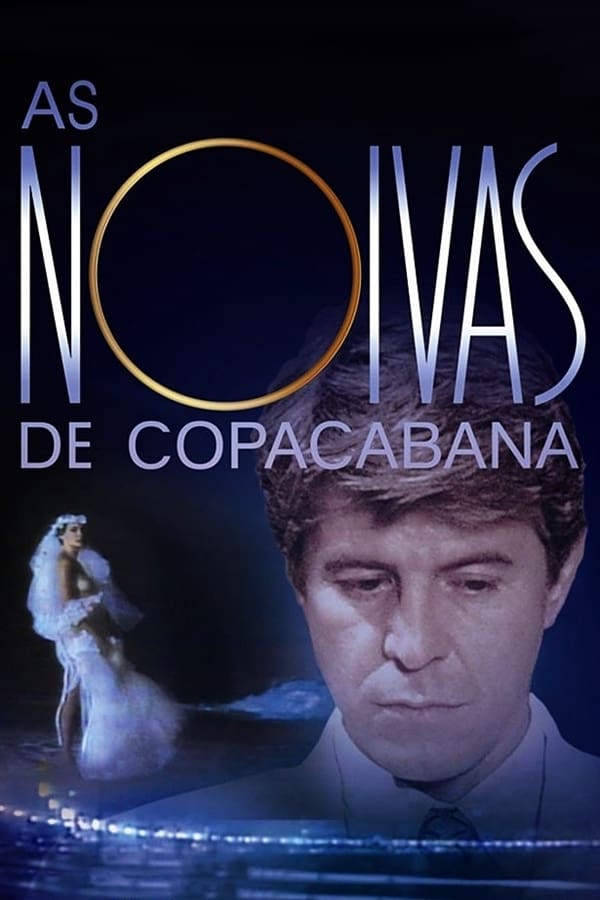The image is a poster or advertisement, featuring a dark background that transitions from solid black at the top to a dark blue at the bottom. Large text spans the top half of the image, starting with "AS" in blue in the top corner. Below, in large, tall letters, it reads "Nuevas de Copacabana," with "Nuevas" in a shimmery silver-blue color and a large "O" resembling a gold moon or ring in the center. The text "De Copacabana" is displayed in a block light blue color.

Central to the image is a man's solemn face with short brown hair, looking downwards to the bottom right. He wears a pale suit, white shirt, and tie. To the left, a woman in a wedding dress and veil stands sideways, looking toward the camera. The background features blue outlines around the man, with hints of city lights below, suggesting a cityscape at night. The overall composition and detailed elements indicate it is likely the front cover of a movie.